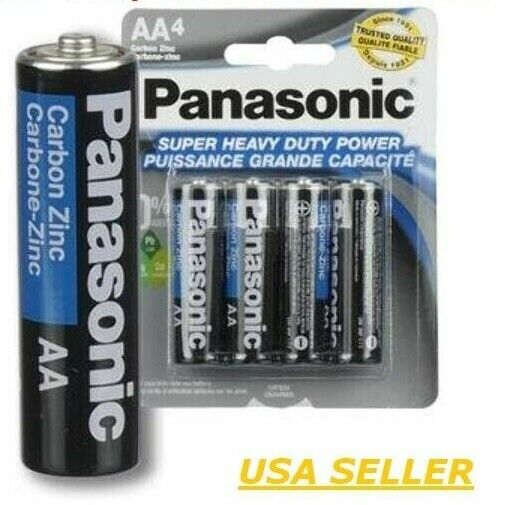The image features a packaging of AA batteries positioned against a white background. The package itself is predominantly black at the top inch, transitioning into a light blue background about halfway down. In the top left corner, in white text, "AA" is displayed followed by a small "4". Beneath this, there are two lines of additional information.

On the right side of this section, there is a yellow circle with black text inside it, and a yellow banner containing two rows of text. Beneath the blue section, "Panasonic" is prominently displayed in white lettering. Above the "Panasonic" logo, there is a small slit for hanging the package on a retail shelf.

The text "Super Heavy Duty power" is written within a blue border, followed by "PUISSANC grande capacité" in white letters. Within the transparent plastic packaging are four AA batteries. Each battery is black with white "Panasonic" lettering, complemented by a blue border and the words "Carbon Zinc," which is also repeated in a foreign language. The batteries feature silver tops and bottoms.

To the left of the packaging is a single AA battery standing upright, identical in design to those in the package. It bears the same silver top, black body with "Panasonic" lettering, and a blue tab indicating "Carbon Zinc." The bottom left of this battery shows the AA size marking.

In the bottom right corner of the image, in bold, all-capital yellow letters with a yellow underline, the text "USA SELLER" is displayed.